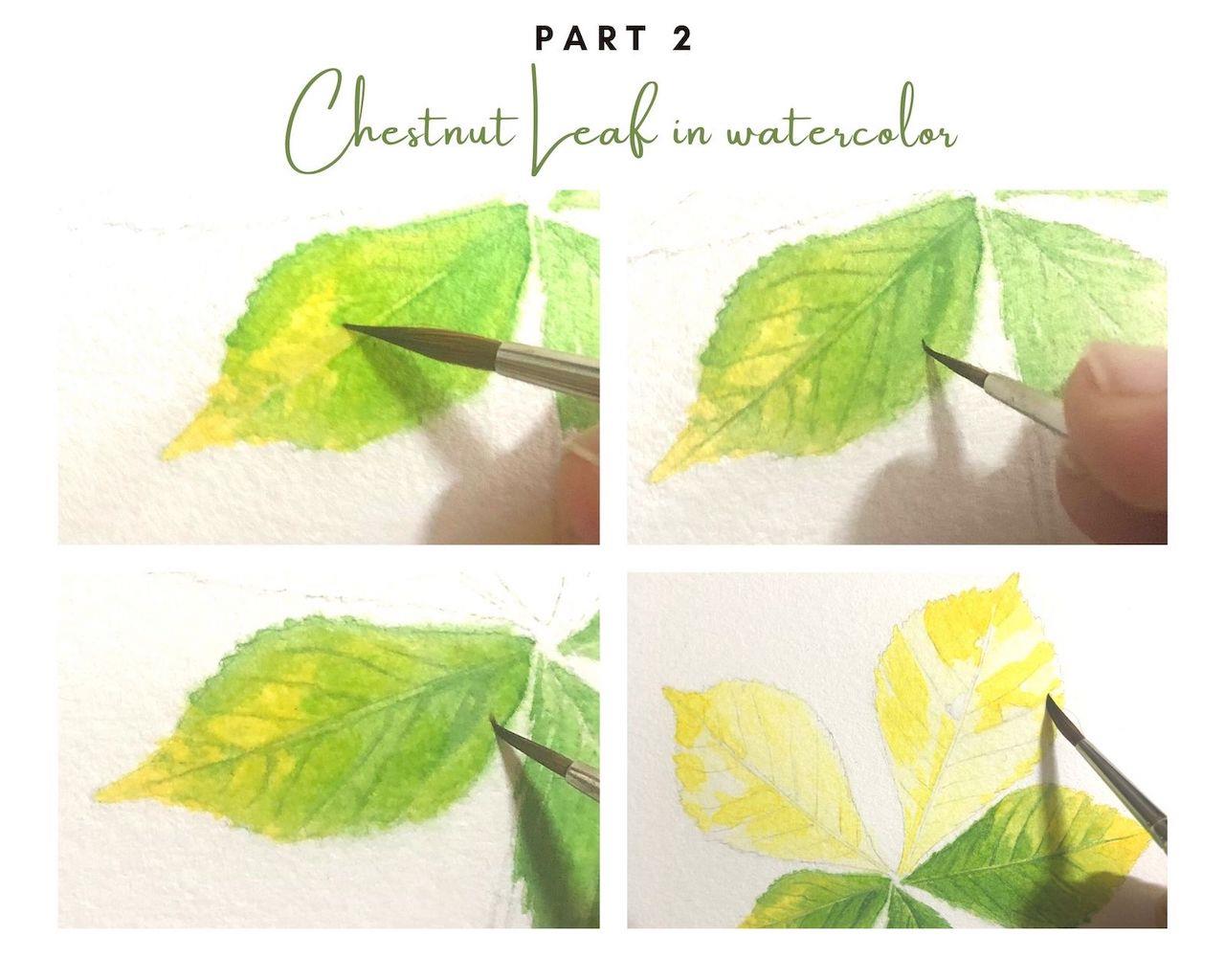This image is an instructional guide titled "Part 2, Chestnut Leaf in Watercolor" and comprises four small rectangular photographs, each depicting a different stage of painting a chestnut leaf. The first panel shows a fine-tipped watercolor brush beginning to fill the outline of a chestnut leaf with green paint. Bright light illuminates the watercolor paper, and the artist's fingertip is slightly visible. In the second panel, the brush is starting to shade the leaf veins, contributing to a darker and more realistic appearance. The third panel highlights the intricate edging of the leaf, with the artist's hand out of the frame, focusing on the intricate detailing. The fourth and final panel reveals the full chestnut leaf, composed of five small leaflets. The lower leaflets are colored in with green, while the upper leaflet remains sketched in pencil with only a yellow base coat applied, indicating the beginning of the final coloring process. The instructional nature of the sequence suggests it could be part of an online watercolor course, showcasing the progressive steps in painting a chestnut leaf from outline to detailed coloration.